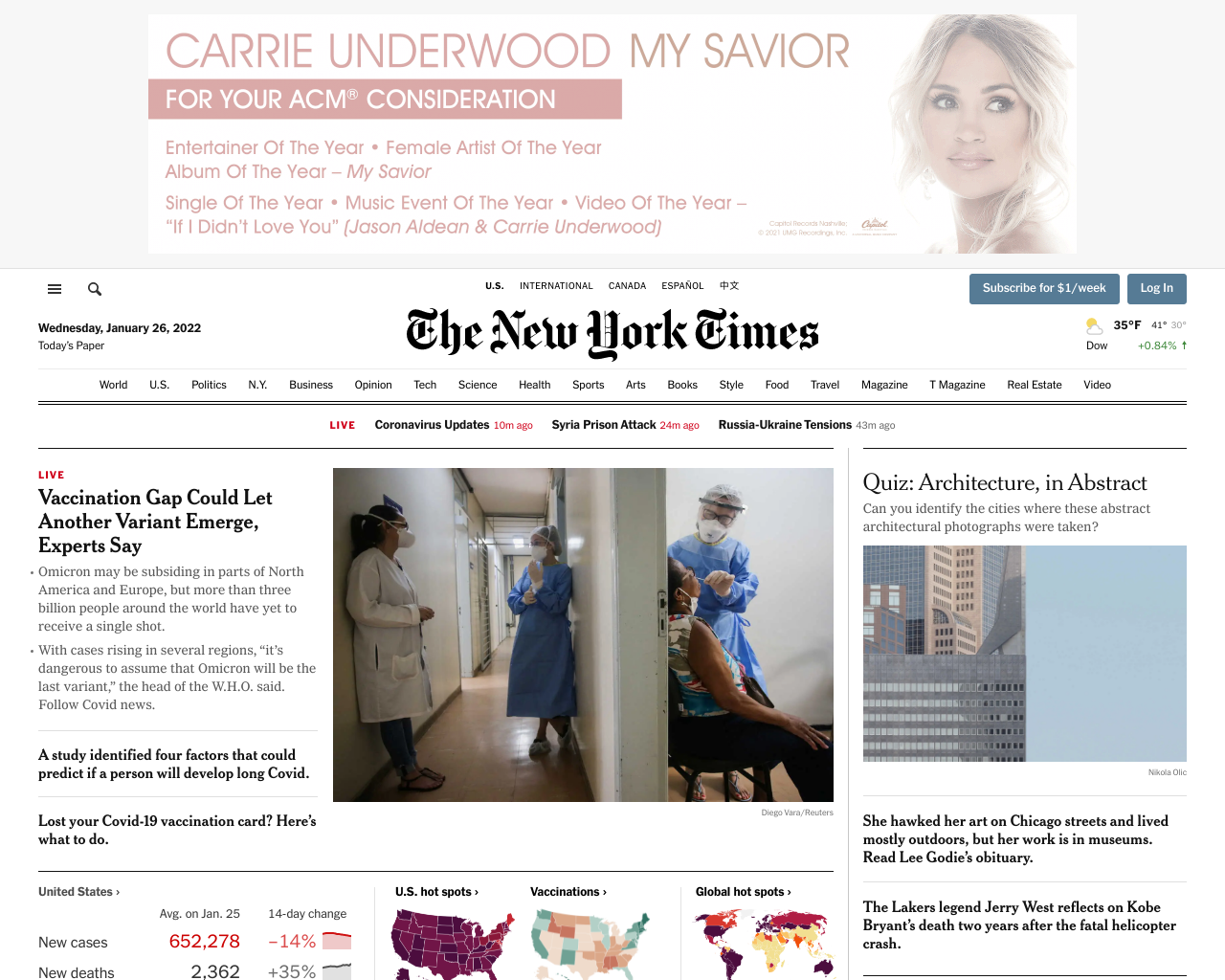The image is a cut-out from the front page of The New York Times dated Wednesday, January 26, 2022. Positioned prominently at the top is an advertisement for Carrie Underwood, promoting her for ACM consideration in categories such as Entertainer of the Year, Album of the Year, and Single of the Year for her collaboration with Jason Aldean on "If I Didn’t Love You." This advertisement includes a picture of Carrie Underwood.

The New York Times masthead is centered in elegant, distinctive typography. Above it, in green text, are options to "Subscribe for a dollar a week" and "Log in."

Below the masthead are the categories: World, USA, Politics, New York, Business, Opinion, Tech, and Science. The main image on this page is a split photograph of two healthcare workers wearing masks, seemingly taken during the COVID-19 pandemic. Part of the image shows a person getting a COVID test from a fully masked and gowned healthcare worker.

Accompanying this image are articles with headlines such as "Vaccination Gap Could Let Another Variant Emerge, Experts Say" and "A Quiz: Architecture in Abstract." At the bottom of the page, there is a map depicting COVID-19 hotspots and vaccination rates globally, alongside statistics of the number of cases and new deaths.

Additionally, on the right side of the page, there is a photograph related to the architecture quiz, showing a large building, contributing to the theme of abstract architecture.